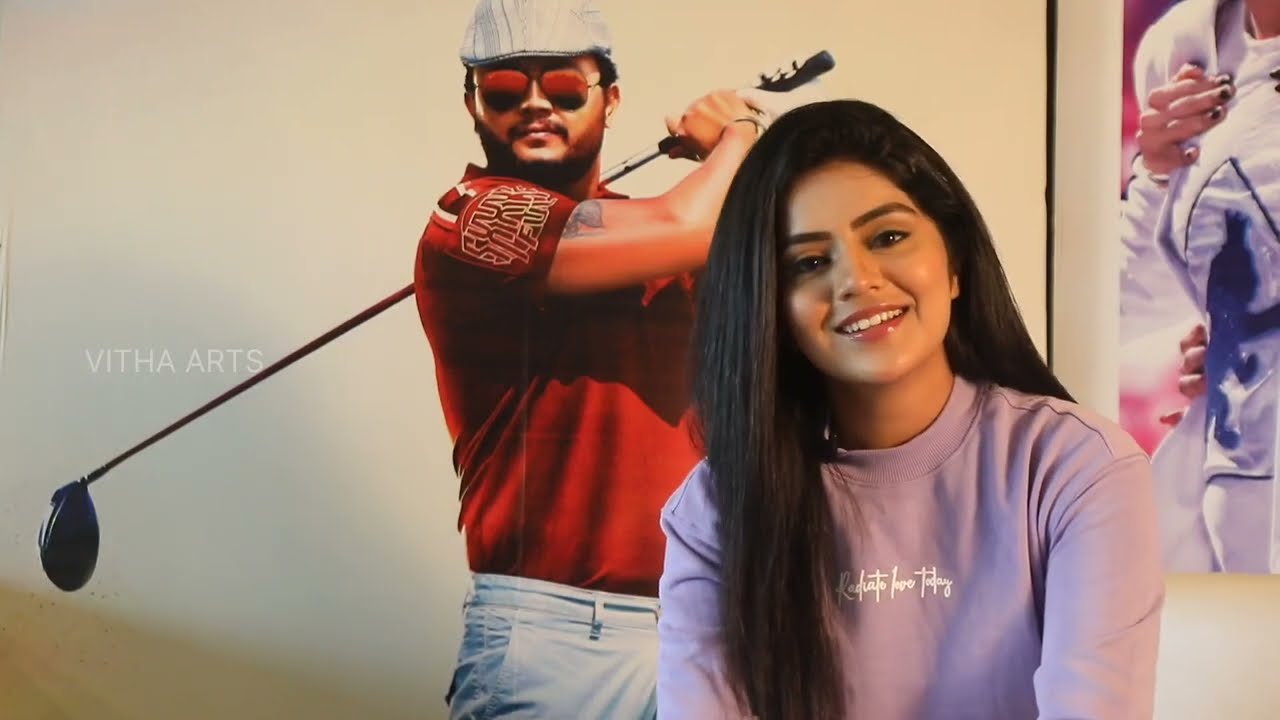The image features a woman with long dark hair, possibly Indian, smiling and looking straight at the camera, showcasing her white teeth. She is dressed in a long-sleeved lavender shirt, which has cursive white text possibly reading "rejoice love today." The shot captures her from the chest up, with her hair parted to the side flowing over her left shoulder. Behind her is a cream-colored wall adorned with a large poster of a male golfer. The golfer, who appears to have just swung his club, is depicted wearing a red polo shirt, white pants, red sunglasses, and a white and black striped golf hat. He holds the golf club behind his shoulder, and to his left, the words "Vitha Arts" are printed in white letters. The overall ambiance suggests an indoor setting with detailed elements highlighting both the woman and the golfer in the background.